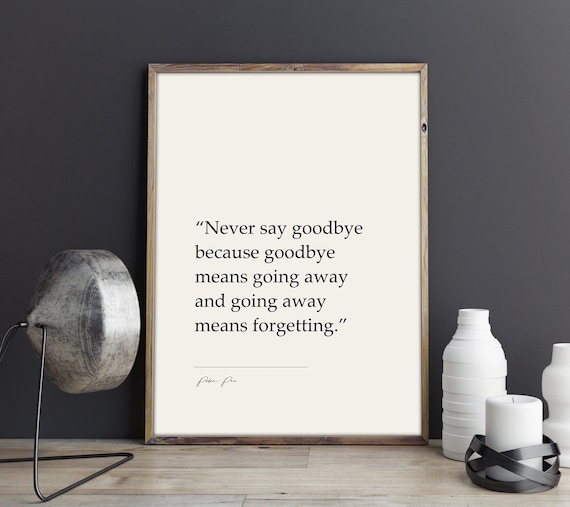In the center of this photograph, a white portrait is prominently displayed against a dark gray wall. The portrait features a poignant quote in black text: "Never say goodbye, because goodbye means going away, and going away means forgetting." Beneath the quote, there is an illegible signature, possibly intended to resemble "Peter Pan." Leaning on a gray, wooden floor that suggests the texture of floorboards, the scene is framed with additional details on either side of the portrait. To the left, there is a distinct silver lamp on a stand, with a visible plug trailing off-frame. On the right side, two white bottles and a white pillar candle in a black, criss-cross metal holder are carefully arranged. The overall composition is visually balanced and evokes a sense of stillness and reflection.